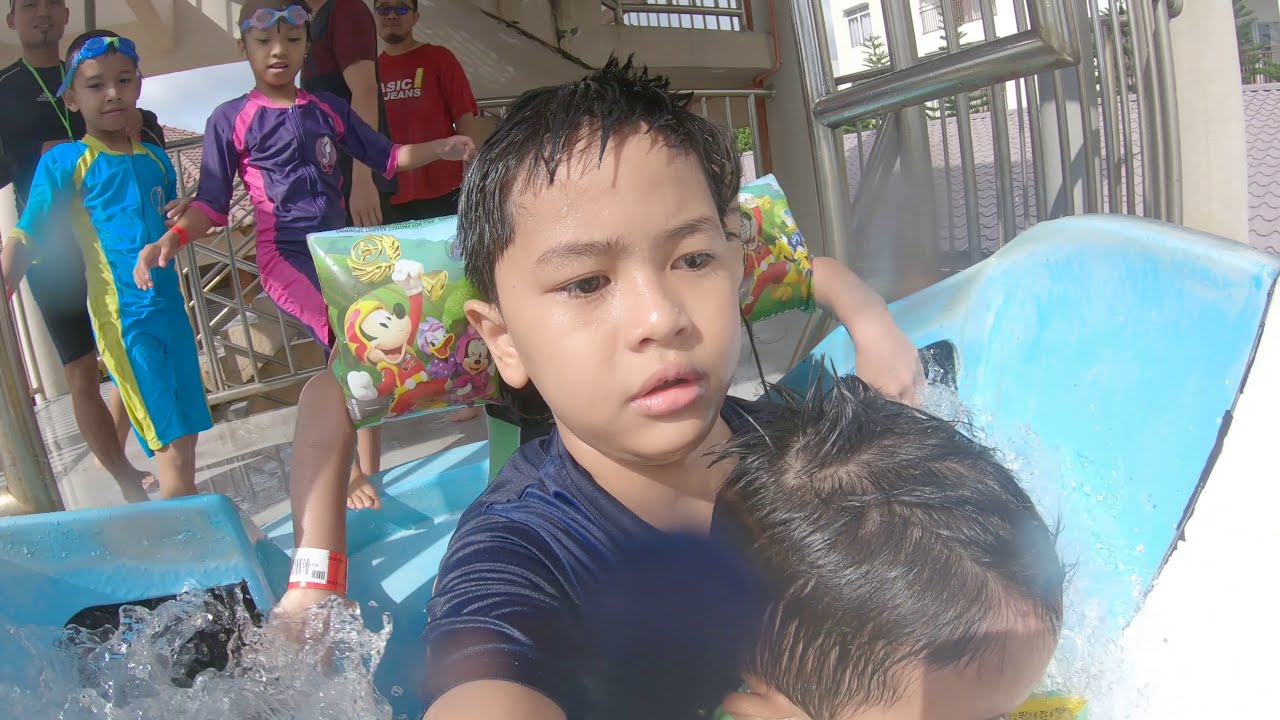This color photograph captures a group of children at a water park, eagerly lined up to go down a slide. Prominently featured at the front center is a young boy with short black hair and brown eyes, wearing a blue (or possibly red) wet shirt, and staring seriously downwards. A smaller child with messy brown hair, parted slightly to the right, is visible in front of him, their head just peeking out.

Directly behind the serious-looking boy, another child is seen with a Mickey Mouse flotation device, showing Mickey holding a gold trophy, and a duck beside him. To the left of this group on a platform stand two more children, both with goggles perched on their foreheads. The child on the left sports a blue suit with yellow stripes, while the one on the right wears a pink outfit with purple stripes. In the background, other young children and several adults, likely including lifeguards, stand observing.

To the upper right, a window reveals an exterior view, showcasing a building with white walls and a tiled roof, separated by a silver barrier. The scene is vibrant, filled with anticipation and the joy of a day spent at the water park.